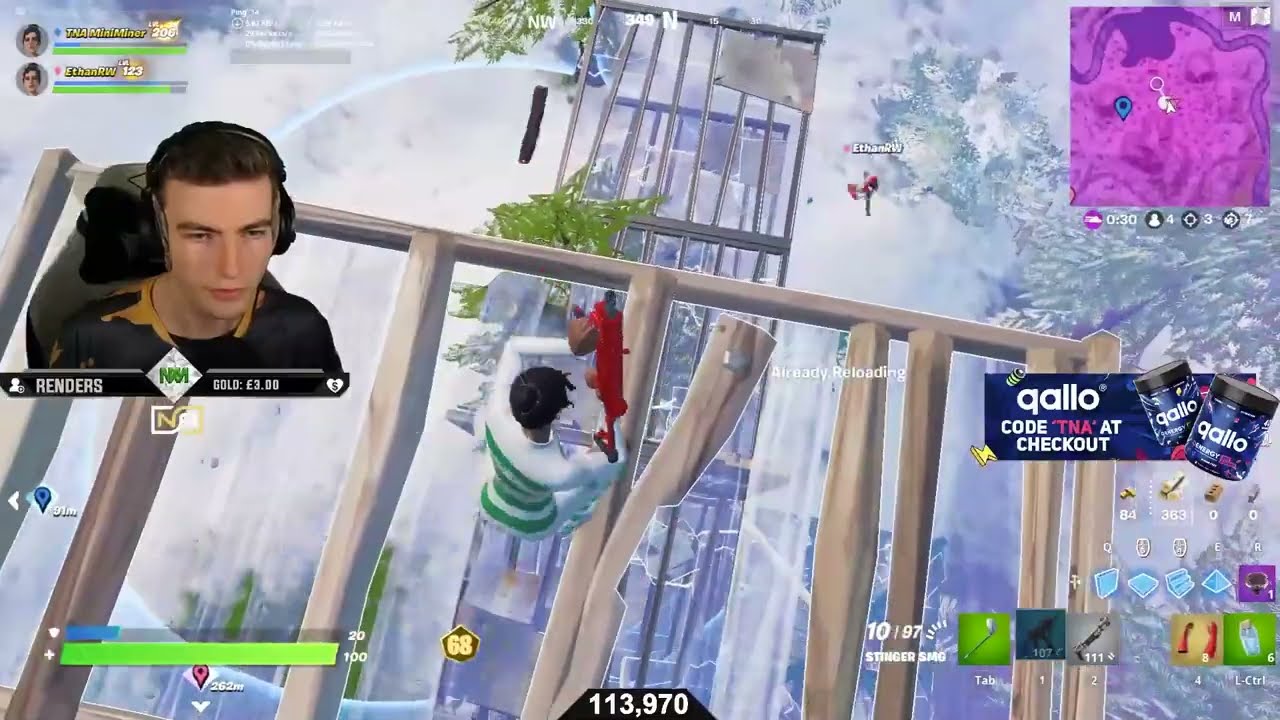In this full-color image, a live stream of a video game is displayed prominently. The scene is split into two main parts: the gamer and the in-game action. To the left, a young Caucasian male, likely in his late teens to early 20s, is wearing headphones and a blue shirt with a yellow collar. His image is overlaid onto the game screen with the text "renders" beneath him, indicating his role as the player.

The game itself is a shooter game viewed from an aerial perspective. The central character in the game, who has dark hair and is wearing a white and green striped shirt, stands on a glass surface bordered by metallic silver beams. This surface is elevated, high above other similar glass structures that are adorned with green plants and shrouded in clouds, with an icy region visible on the right side of the sky.

The character holds a red weapon and appears in a precarious position high above the rest of the game environment. Technical elements include a purple map indicating the character's location in the upper right corner, and a scoreboard displaying "113,970" at the bottom middle of the screen, likely representing points or coins. On the bottom right, there is a game menu featuring various controls labeled "1, 2, 4," and other options necessary for gameplay.